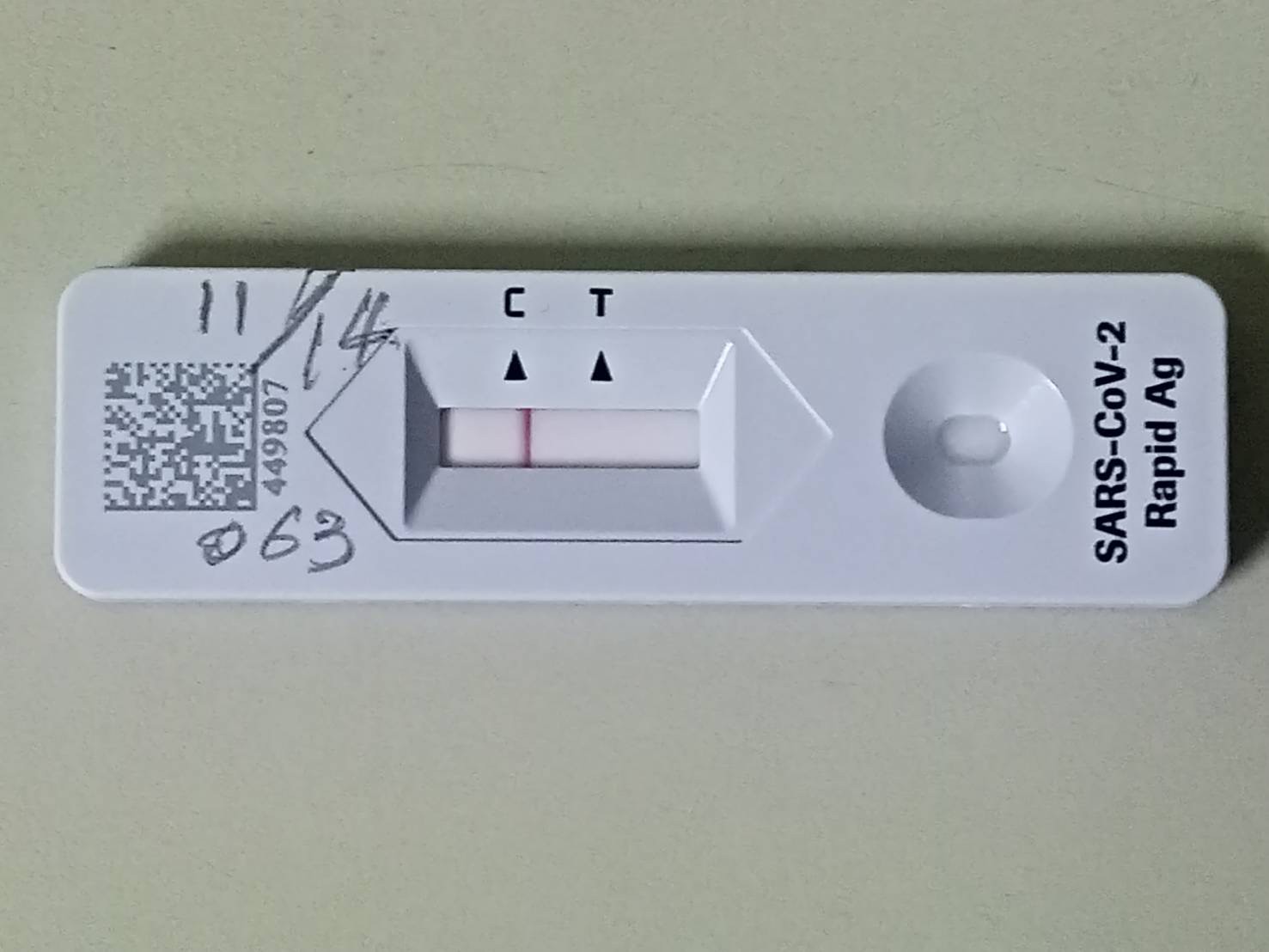This photograph showcases a rectangular medical testing device prominently labeled "SARS-COV-2 Rapid AG" on the right-hand side, indicating it is designed for COVID-19 testing. A scannable QR code is located on the left-hand side of the device, accompanied by the number 449807. Just above the QR code, there are handwritten annotations reading "11/14" and below, "063". 

In the center of the device, there are two labeled sections for reading the test results: "C" on the left and "T" on the right. The right-hand end of the device features a small receptacle designated for the liquid sample drop. The overall layout and markings on the device are indicative of a rapid antigen test designed for quick and efficient COVID-19 detection.